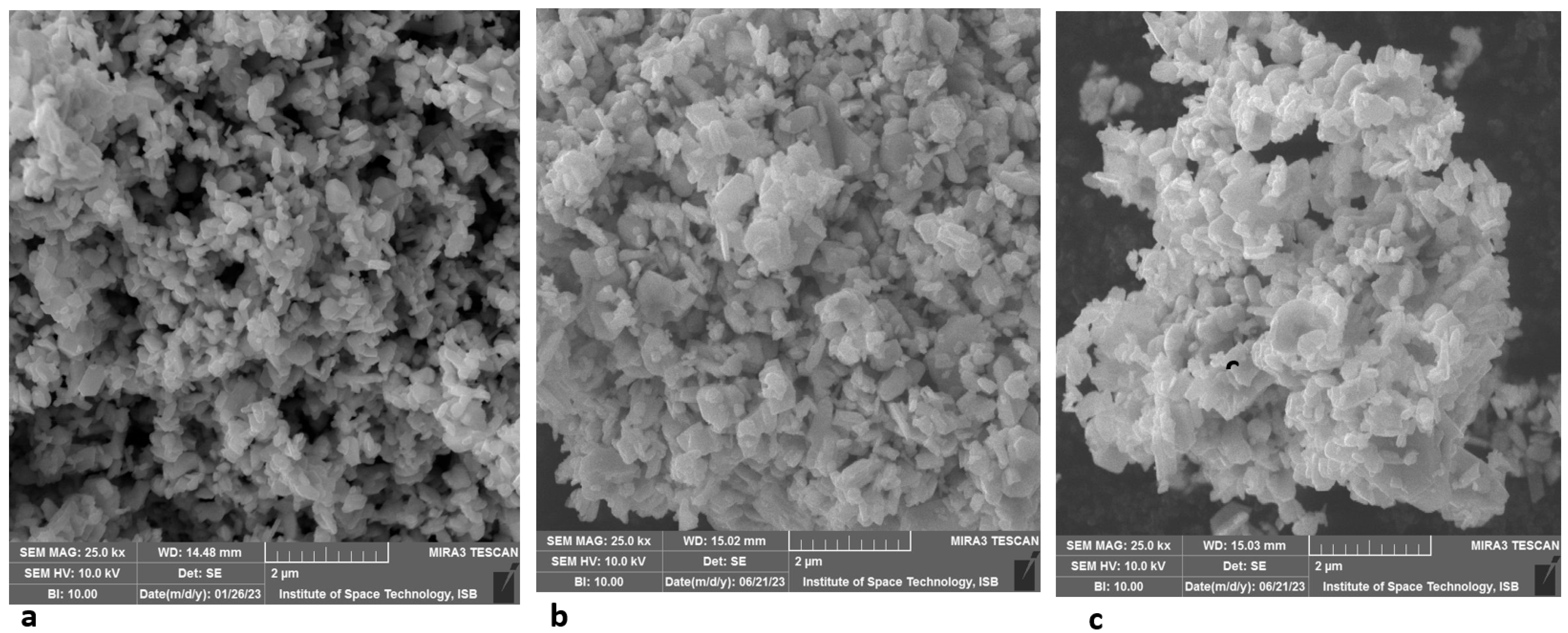The three black and white images from the Institute of Space Technology depict microscopic views of various clumpy substances or growths, each measuring approximately 14-15 millimeters in width. These high-resolution scans, as indicated by details such as "SEM mag 25.0 kx" and "SEM HV 10.0 kv," show grainy, textured materials that resemble piles of rice, sand, shavings, or potentially biological entities like bacteria or maggots. Each image includes a detailed menu at the bottom displaying technical specifics: magnification levels, working distance (WD 14.48 mm), and the scan date (126.23). Despite the varied positioning and forms of the materials, all three images maintain a uniform size and perspective, highlighting the subject under microscopic examination. The exact nature of the substances remains ambiguous, adding a layer of intrigue to these detailed scientific captures.